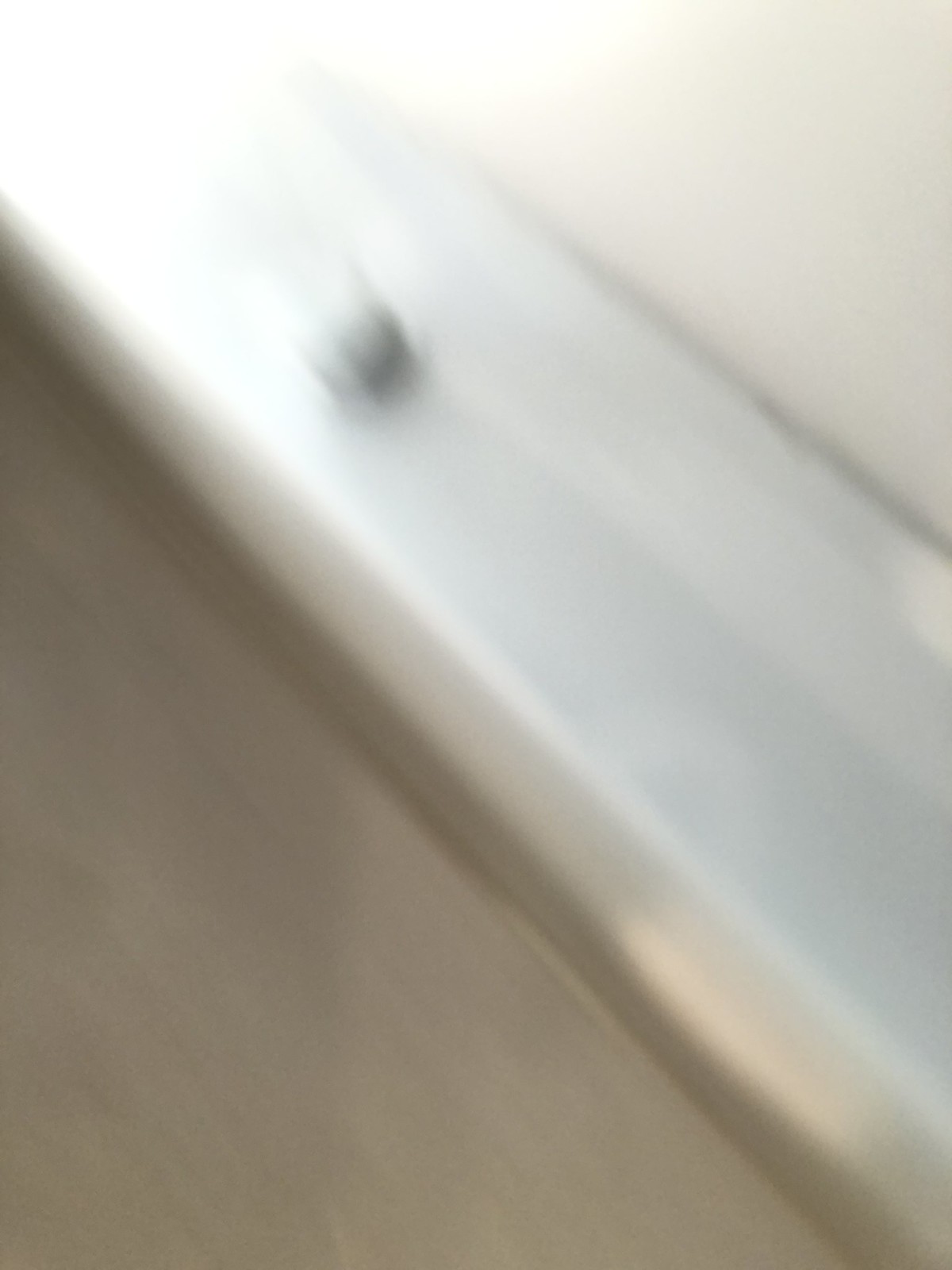This is a colour photograph characterized by significant blurriness, rendering the subject indistinct and challenging to identify. In the top left corner, there is a white light that dominates the upper portion, causing an overexposure effect and obscuring the surrounding details. Below the light, there is a vaguely defined triangle in shades of beige and grey. Cutting diagonally across the photograph is a prominent beige line with a small, metallic-edged round object at its center. Towards the bottom edge of the line, a hint of gold glimmers. Adjacent to this line is another triangular shape, which features dark brown and gold hues. The overall composition appears to mimic the outline of a bathtub, with the metallic object resembling a plug, although no taps are visible. The perspective is skewed, imparting an unnatural, diagonal orientation to the elements within the frame. The image lacks other discernible features, contributing to its abstract and ambiguous nature.